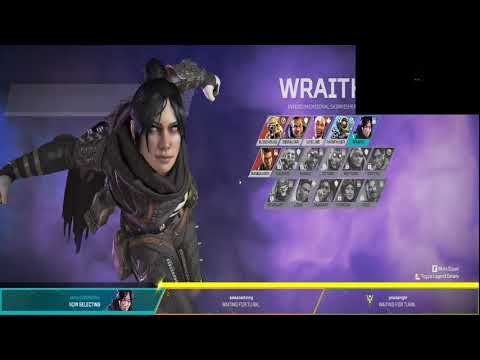The image is a screenshot from the video game "Apex Legends" showing the character select screen. Dominating the left side is a woman named Wraith, identified by the white text at the top center. Wraith is dressed in an all-black outfit, including a leather jacket, scarf, and pants. Her black hair is swept up in a bun, and she has distinctive white eyes with black makeup around them, giving her a tough, intense look. The background is a hazy, smoky purple, adding an eerie ambiance to the scene. To the right, we see a grid of sideways slanted squares displaying various characters, many of which are grayed out and locked. At the bottom, there are colored rectangles, yellow, purple, and teal. The screen seems to be partially overlaid by a blank black square on the top right, possibly a space for a live stream or video. Overall, this detailed screenshot captures the essence of the character selection in "Apex Legends," focusing on the enigmatic character Wraith.